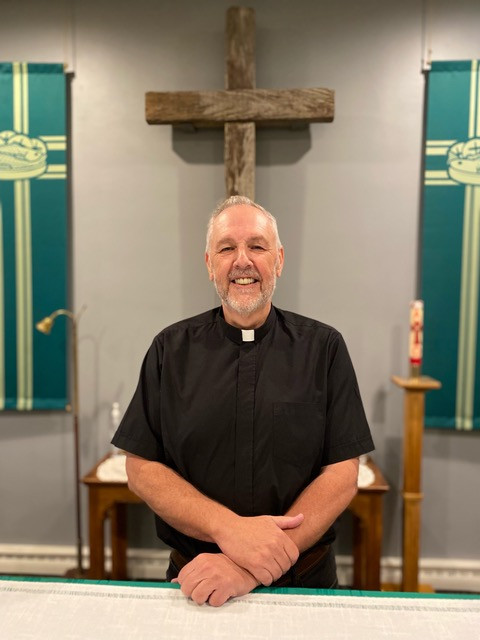This photograph, presented in portrait layout, features a middle-aged Caucasian man, presumably in his fifties, identified as a priest. He sports a short, gray, balding hair, alongside a gray stubbly beard and mustache. He is dressed in a traditional short-sleeved black clerical shirt with a white collar insert, indicative of his religious vocation, possibly as a Roman Catholic or Episcopalian priest. The priest stands at a white counter with a green border, smiling warmly with folded arms.

In the background, an austere wooden cross hangs on a gray wall, seeming to emerge just above his head. Flanking the cross are two seafoam green banners, each adorned with yellow markings, resembling a cross and potentially a crown of thorns design. Also present in the background is a wooden altar, a pedestal with a red candle, and a tool likely used for candle snuffing. The setting appears to be a small church, evoking an intimate and devout atmosphere, with the priest radiating a sense of contentment and joy.